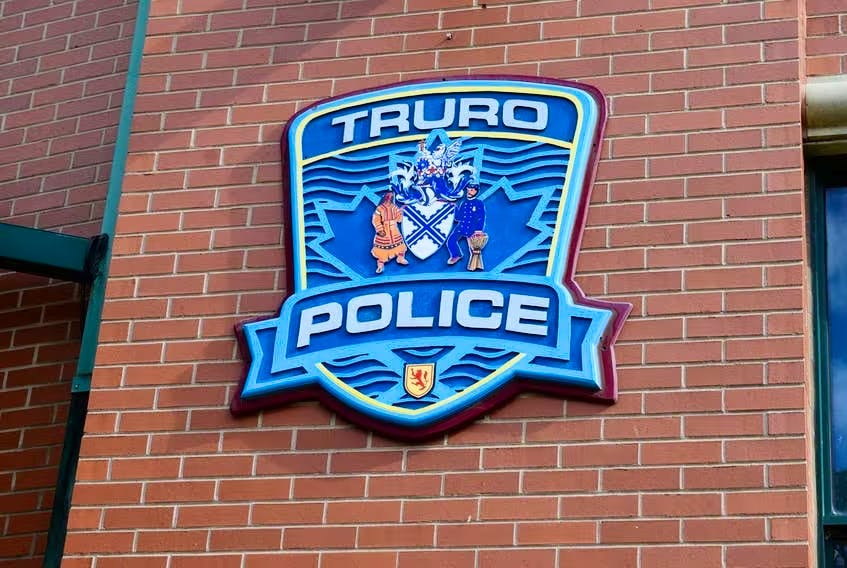The photograph showcases the exterior of a police department building constructed with red brick. Prominently displayed in the center of the image is the emblem of the Truro Police, outlined in dark red. The emblem features a dark blue background with a contrasting light blue trim and includes elements such as a Canadian maple leaf, a Native American figure on the left, a police officer on the right, and a blue and white shield with an X in its center. Above the shield, intricate design work is visible, while a smaller shield with a yellow background and red line is situated below. The building's brickwork is reflected in a glass window, creating a mirrored effect. Additionally, the left side of the image includes a vertical metal pole, adding to the architectural details of the police office setting.